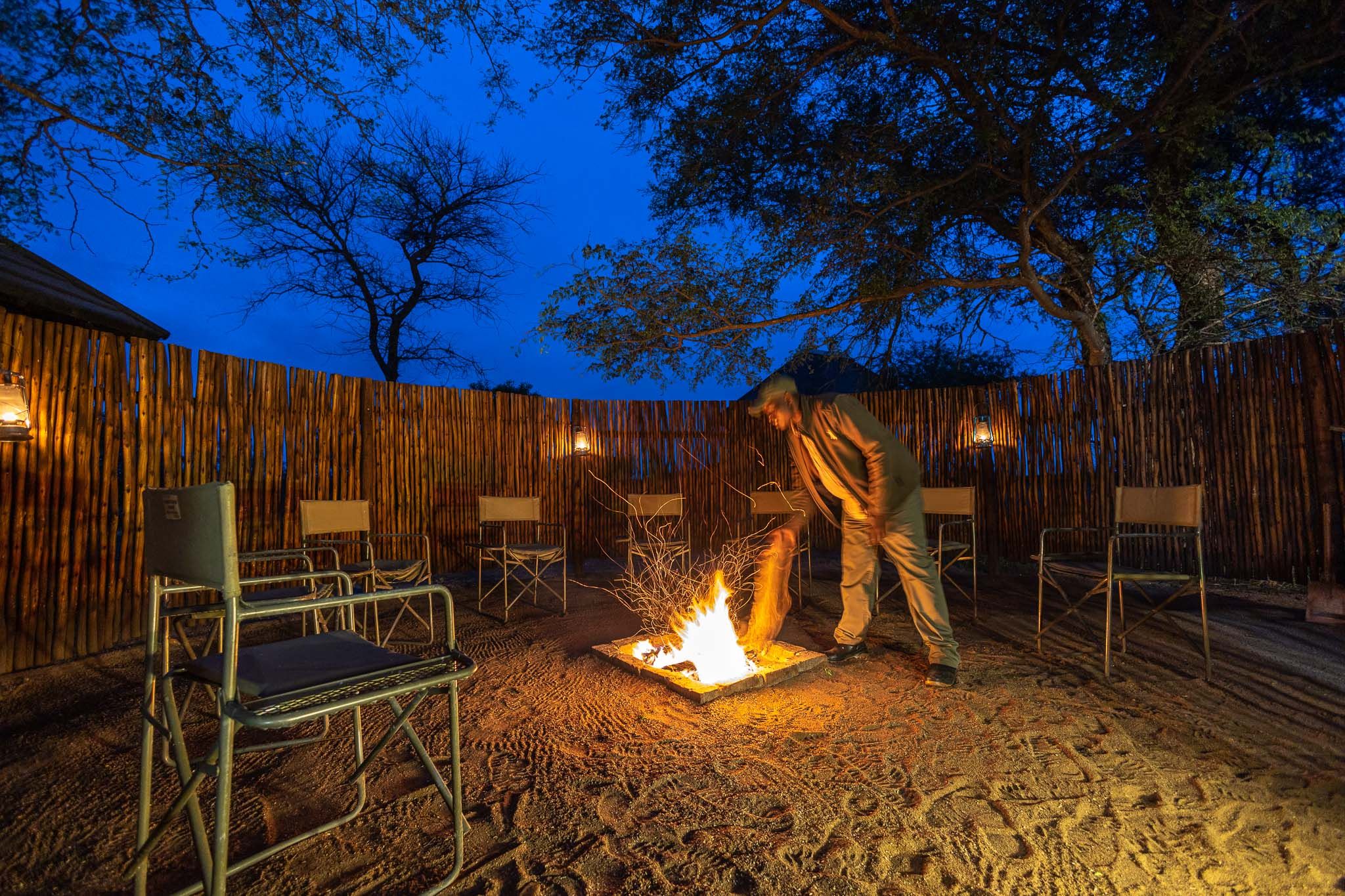This nighttime photograph captures a serene outdoor scene with a clear dark blue sky overhead. At the heart of the image is a campfire, its flames casting a bright orange glow that contrasts with the dim surroundings. A man, dressed in a tan hat, brown jacket, and tan pants, stands beside the fire, seemingly adding a log to it. The area around the fire pit is sandy, reminiscent of a beach, and is dotted with various footprints. Encircling the campfire is a semicircle of eight empty chairs, inviting future gatherings.

In the background, the yard is bordered by a bamboo or wooden stick fence, which curves around the scene. Along this fence, three lanterns provide additional dim lighting. Behind the fence, a few trees are silhouetted against the dusky sky, adding a touch of natural beauty. To the left of the image, there's a glimpse of a neighboring house's roof, hinting at the location being part of a residential area. This detailed composition combines elements of nature, human presence, and subtle lighting to create a tranquil nighttime vignette.